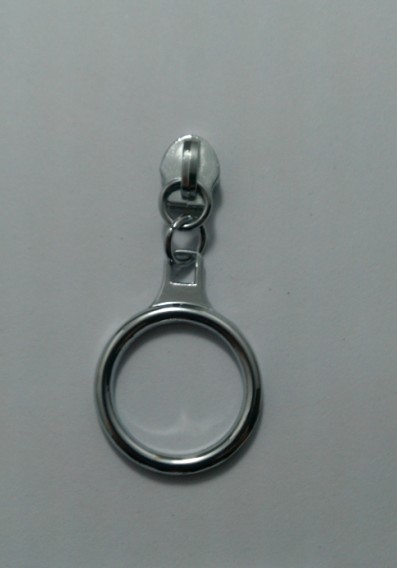The image depicts a close-up of a zipper pull, light gray in color, resting on a gray surface. The zipper pull features two small chain links attached to it, with the bottom link connecting to a key ring, which serves as the pull mechanism. Light shines from above, creating a bit of shadow at the base of the key ring and underneath the zipper pull. There is also a delicate shine on the top of the zipper pull and the inner and outer top edges of the key ring, highlighting its details against the gray background.